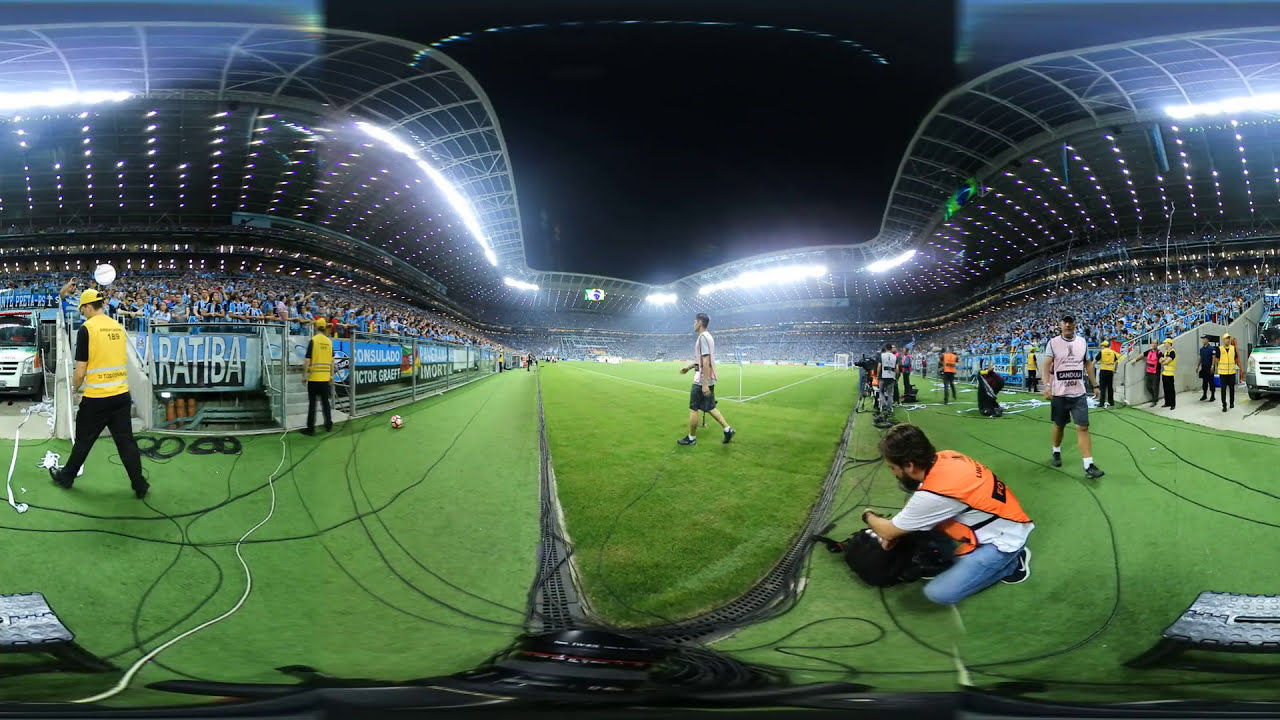The image captures a panoramic view of a nighttime soccer match in an arena, depicted through a series of interconnected, slightly warped photographs, possibly taken with a fisheye or 360-degree lens. The crowd, dressed predominantly in light blue, fills the bleachers surrounding the brightly lit grass field. Several officials, identifiable by their black attire with bright yellow tops, stand along the edges of the field, facing the audience. Prominently, a soccer player donning a short-sleeved shirt and shorts is captured mid-stride in the center, heading towards the left side of the image where a soccer ball is visible. On the lower right, a cameraman in an orange vest is seen squatting, intently focused with his camera aimed at the field. The image conveys a dynamic and somewhat surreal atmosphere due to its visual distortion, integrating multiple perspectives into one cohesive panorama.